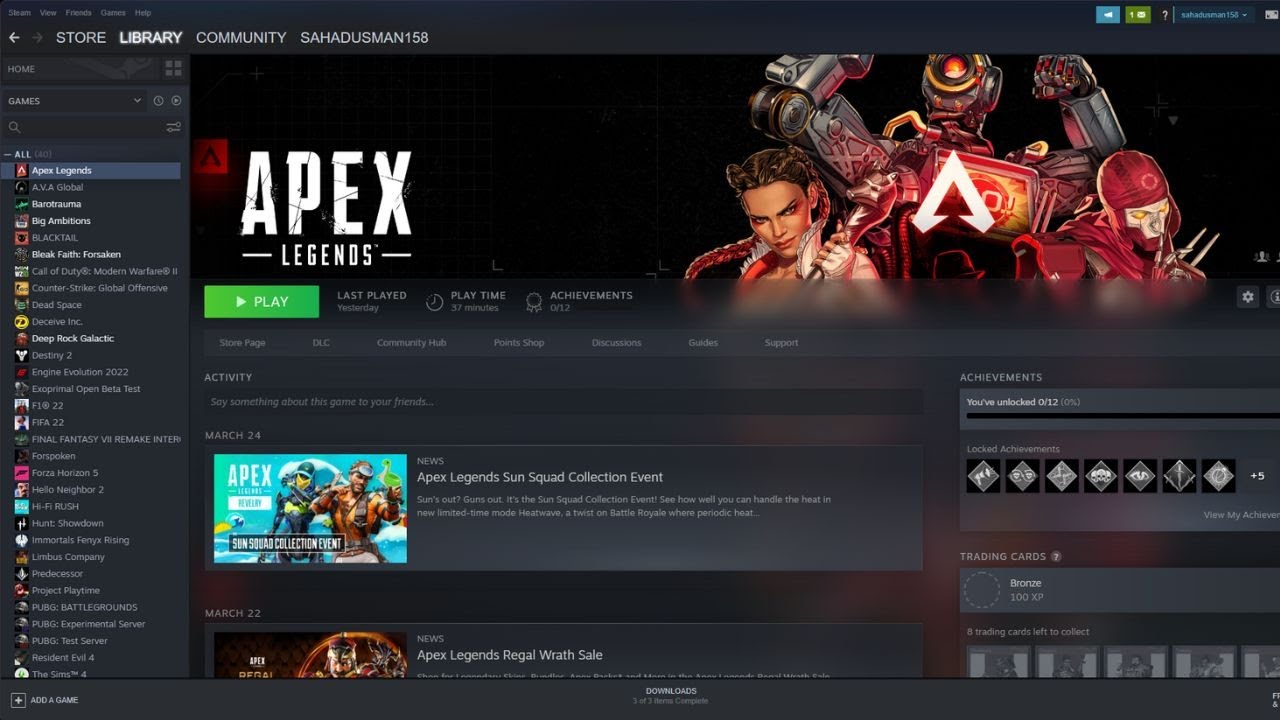The image depicts the homepage of a gaming website featuring "Apex Legends." The background is predominantly black, providing a sleek, modern interface. At the top of the page, navigational tabs read "Store," "Library," and "Community," with the username "Sahazman 158" displayed prominently. 

Illuminated text highlights the "Library" section, creating a focal point. The right-hand corner of the screen displays a blue health bar, a green shield bar, and additional greenish-blue text, perhaps indicating in-game statuses or online indicators. 

On the left side, a vertical menu lists various video games, offering a plethora of choices for the user. While not fully familiar with Apex Legends, the user notices a green "Play" button underneath the title, inviting interaction. 

The middle section showcases vivid, dynamic images from the game, featuring three characters: a female warrior, a male suited in high-tech armor, and another male wearing a mask paired with armor. The Apex Legends logo in blue dominates the center, with images of two game characters prominently displayed. A glimpse of a third character is partially visible at the bottom, cut off by the screen edge. This detailed composition highlights both the aesthetic appeal and the interactive elements of the gaming webpage.